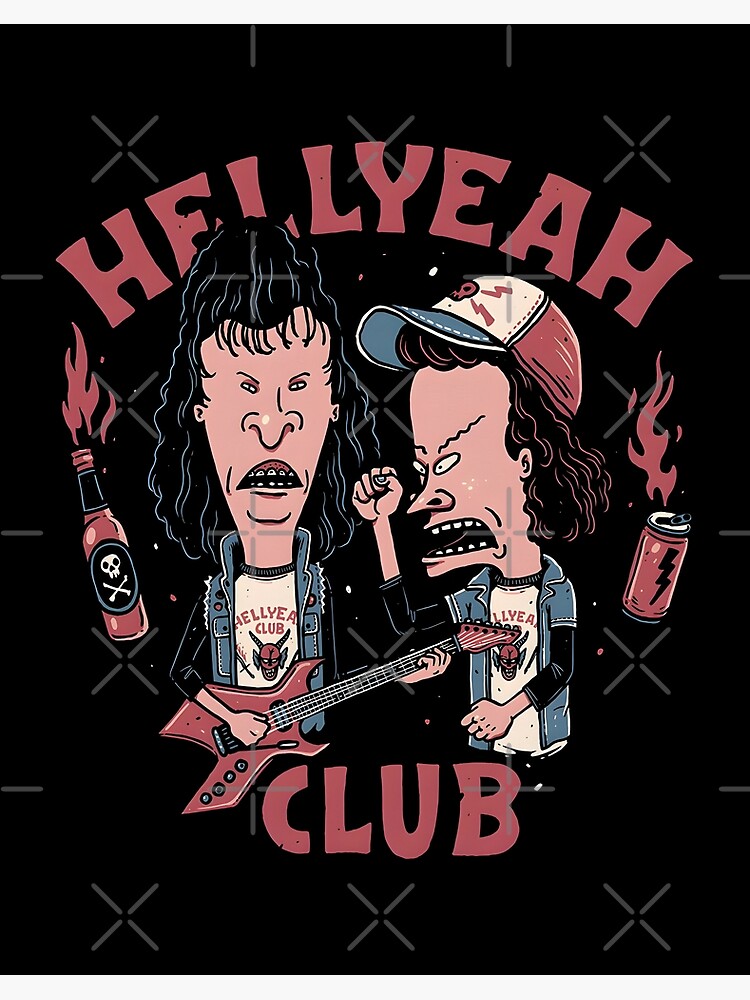This animated image of Beavis and Butthead appears to be styled as a poster on a black background adorned with a pattern of alternating rows of X's and lines. At the top in bold, red letters, it reads "Hell Yeah," followed by "Club" underneath. Beavis and Butthead are positioned centrally, both clad in jean jackets with black sleeves, wearing white T-shirts that read "Hell Yeah Club" with a devil graphic below the text. The character on the left, holding an electric guitar, stands next to a flaming beer bottle marked with a skull and crossbones. To his right, Butthead—distinguished by his hat adorned with a skull and lightning bolts, and longer hair—raises his fist angrily towards Beavis, with his mouth open as if shouting. On the far right, a flaming beer can with a lightning bolt is also depicted.